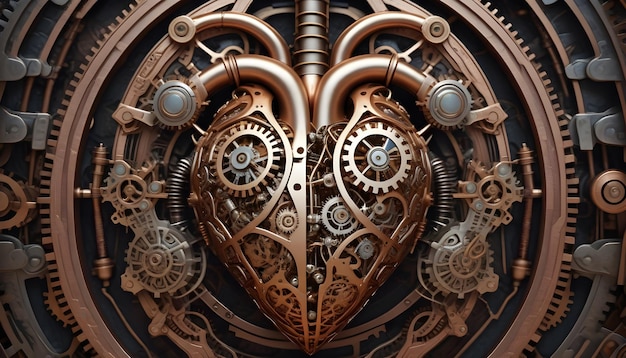This intricate image portrays a steampunk-inspired mechanical door, meticulously crafted from interlocking gold, silver, and bronze components. Dominating the center is a heart-shaped handle flanked by prominent gears, emblematic of the door's elaborate design. The heart, tinged with faint reddish-brown and subtle hints of dark green, melds seamlessly into the composition, highlighting the detailed craftsmanship. Surrounding the central heart are numerous smaller mechanical parts, including spoked circles and grommets, which suggest movement and complexity. The overall scene evokes the aesthetic of an ornate piece of machinery, with its filigree-like metalwork contributing to a richly textured and visually captivating image.